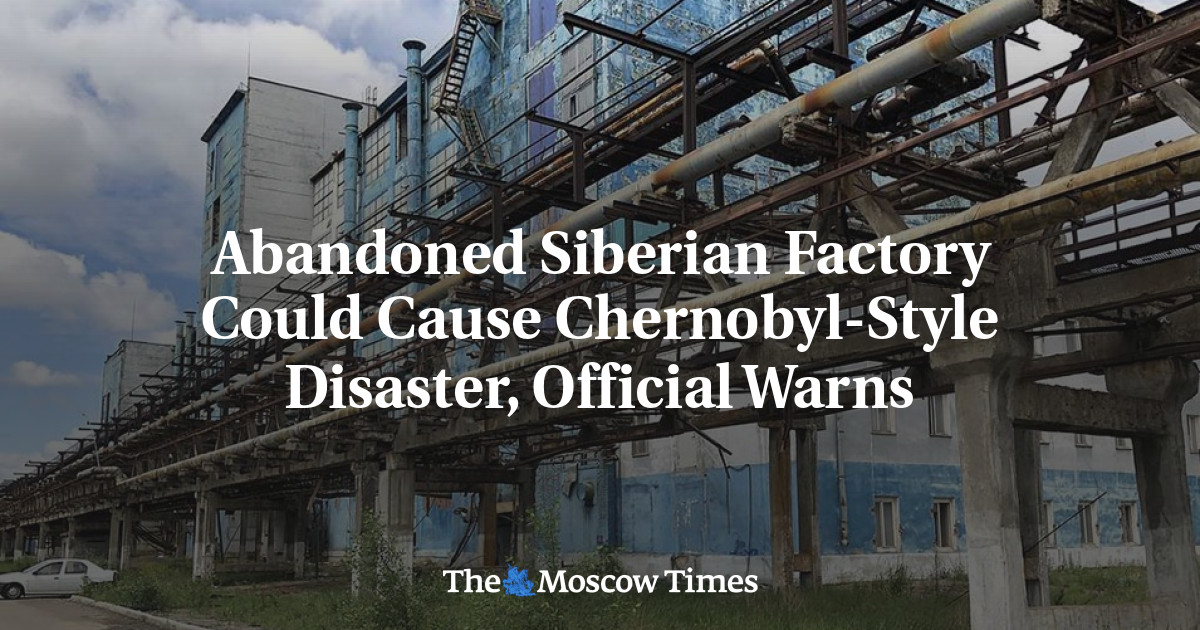The image, a horizontally aligned rectangle, prominently features an old abandoned factory at its center. The factory, made of gray and white stone, exhibits signs of neglect with its surrounding bars, wires, and an unfinished bridge structure in the foreground, supported by large cement blocks. Smokestacks emerge from the factory, accentuating its industrial nature. A small patch of grass grows in an open lot below the factory, indicating further signs of disuse. On the bottom left corner, a white compact sedan is parked beside a curb in a small parking lot. The background transitions to a partly cloudy blue sky in the top left, which provides a stark contrast to the dilapidation below. Superimposed over the center of the image in white text, it reads: "Abandoned Siberian factory could cause Chernobyl-style disaster, official warns." Below this text, smaller white lettering at the bottom says, "The Moscow Times." This image likely serves as a cover for an article warning of potential industrial disasters similar to Chernobyl, highlighting the grave concerns officials hold over the site's current state. The colors in the image range from the grays and whites of the factory and the brown of the structural bars to the greens of the grass and the blues and whites of the sky.